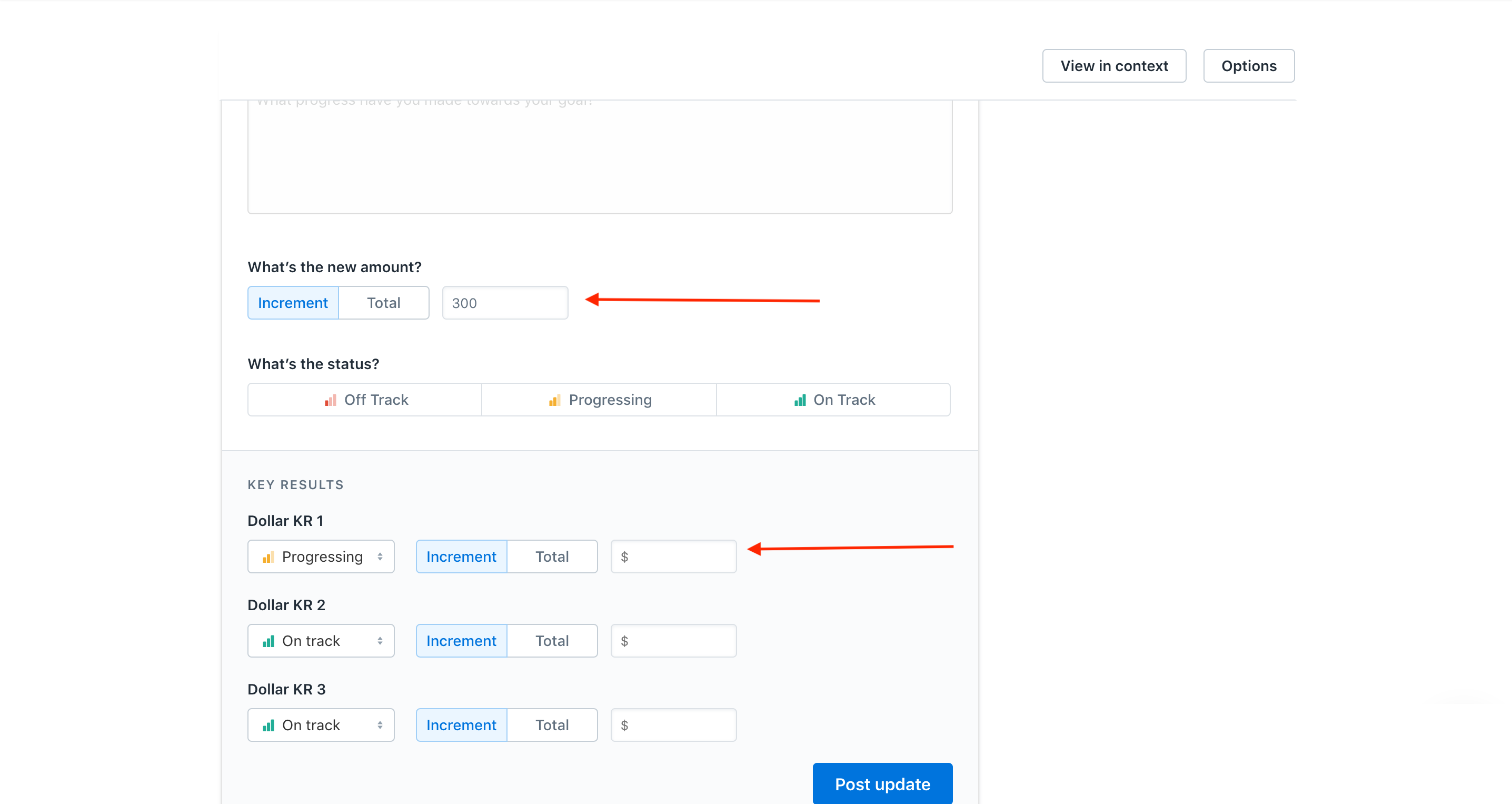In this image, we see a screenshot set against a solid white background featuring a user interface with a clean and structured layout. At the top of the interface, a rectangular box is outlined in light gray. Below this box, on the left side, bold black text asks, "What's the new amount?" Immediately beneath this query, the word "Increment" is displayed in blue text. Adjacent to the word "Increment," on the right side, is the word "Total" in gray text. Positioned below these labels is another box displaying the amount "300," which is highlighted by a red arrow pointing directly at it.

Further down the interface, the section is titled with bold text asking, "What's the status?" Directly underneath this question, three boxes appear consecutively from left to right labeled "Off track," "Progressing," and "On track."

The subsequent section is labeled "Key Results" and lists the following details in sequence:
- "$KR1, progressing increment total."
- "$KR2, on track increment total."
- "$KR3, on track increment total."

In the bottom right corner of the interface, there is an action button colored in blue with the white text "Post Update," designed to facilitate user interaction.